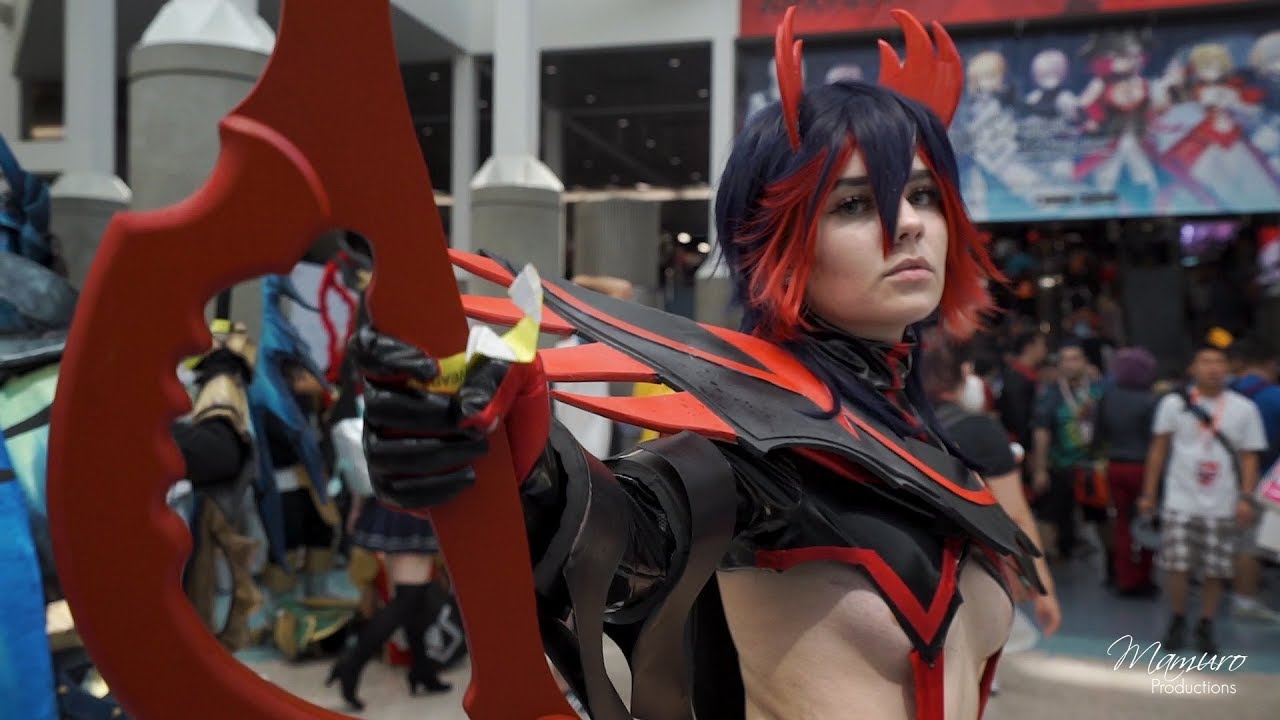The photograph depicts a young Caucasian woman cosplaying as a character from the anime "Kill La Kill" at what appears to be a convention, possibly Comic-Con. She has a dark bob haircut with red and blue tips and adorns fire-like horn decorations on her head. Her outfit includes a striking combination of black and red elements, featuring a black shield-like accessory extending from her chest with red spikes. Her right arm is fully covered in a black sleeve adorned with black gloves, and she's holding a large red weapon resembling the blade of a pair of scissors, a distinctive attribute of the character she is portraying. The costume is somewhat revealing, with minimal fabric covering her chest. The background shows a blurred crowd, with some attendees in various costumes and others in regular attire, emphasizing the bustling, vibrant atmosphere of the event. The bottom right of the image is marked with the text "Memuro Productions," where "Memuro" is styled in cursive white and "Productions" in plain white. The woman is looking directly at the camera, capturing a sense of intensity and engagement in her performance.